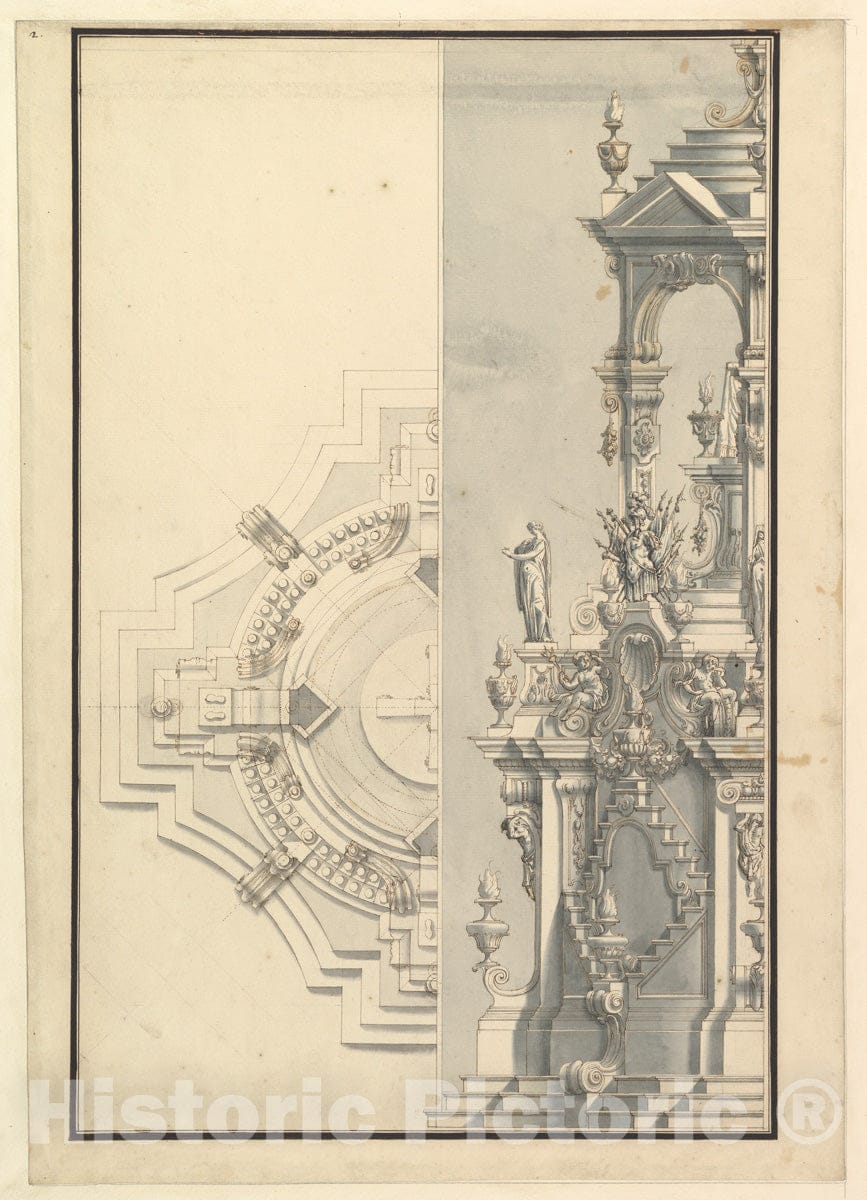The image features an aged, yellowed piece of paper used as a background. This paper seems to be an old, worn-out type with a cream to grey gradient. At the bottom of the image, there's a watermark saying "Historic Pictoric" with a copyright symbol next to it. The image is divided into two panels: the left panel depicts a bird's-eye view of a multi-level architectural platform or stage, featuring a circular cross in the center and light grid lines sketching out the details. The right panel, set against a darker grey background, shows a side view of an ornate stone monument adorned with intricate carvings, patterns, and several statues. One prominent figure appears to be a woman with wings. The elaborate and detailed nature of the drawings suggests that these might be plans for a significant historical or commemorative structure.